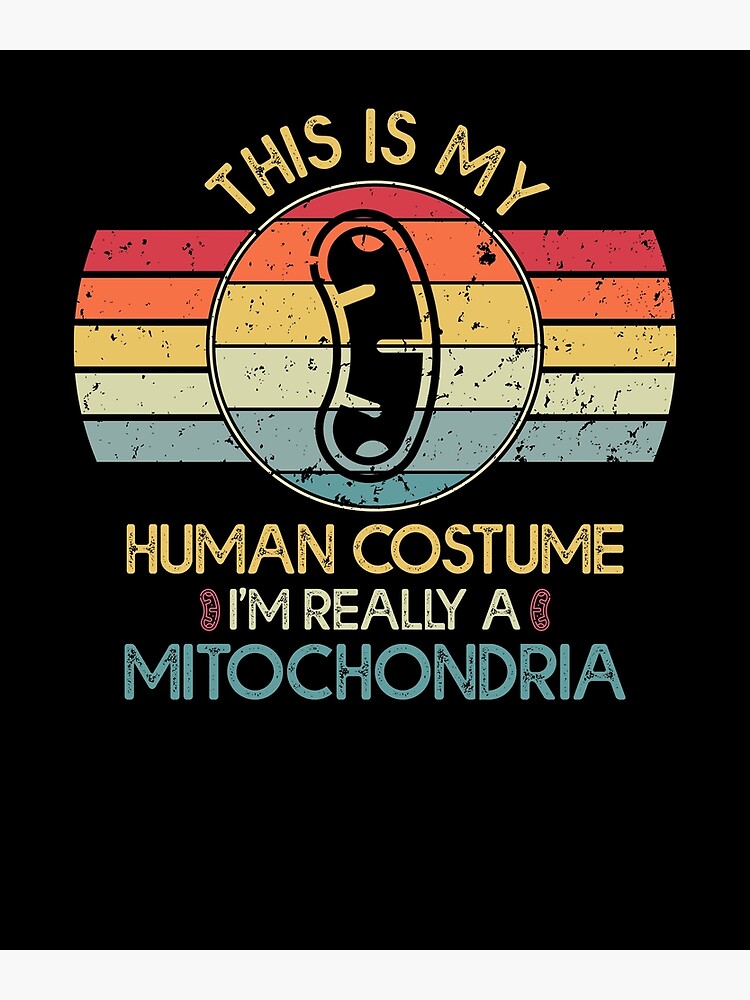The image is a rectangular poster or graphic design, possibly for a t-shirt, with a height-to-width ratio of 1:2. It features a thin gray border along the top and bottom edges. The background is noticeably black. In the center of the image, there is a design comprised of a colorful element and various text inscriptions. At the top of the design, bold yellow text reads, "this is my". Below it, there is a vibrant illustration with lines in red, orange, yellow, green, and blue, converging into a circle at the center. Within the circle, there's a bean-shaped black outline, representing a mitochondria, although its initial appearance could be mistakenly identified as a hot dog or jelly bean. Underneath this graphic, more yellow text reads "human costume". The text continues below in white, stating "I'm really a", and concludes in light blue text at the bottom with the word "mitochondria". The entire image carries a stylized, worn look, emphasizing its casual and humorous theme.